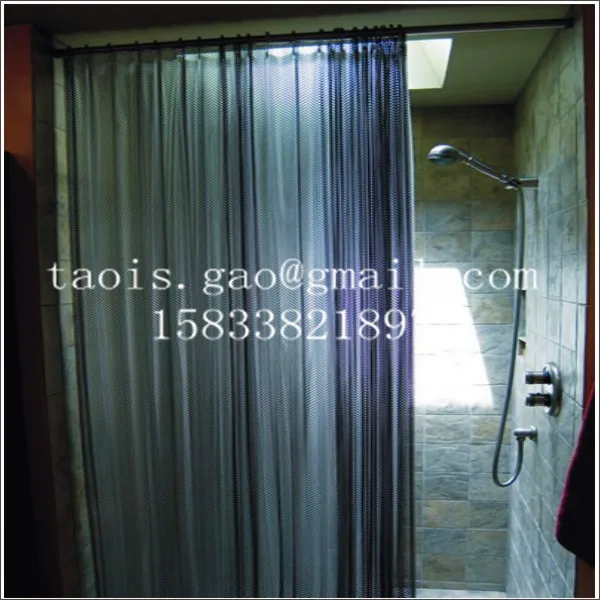The image captures a walk-in shower with rather dark lighting. Dominating the scene is a shower curtain, hanging from a rod across the middle to the left side of the photo, displaying shades of blue, gray, and purple. The background reveals a stone-tiled wall featuring a mixture of tans, browns, and grays. On the upper right side, a silver shower head is mounted, connected via a long cord to two silver handles below. There is visible light reflecting off the ceiling from a skylight above the shower. The bottom edge of the photo shows a glimpse of the tiled floor. Prominently overlaying the center of the image is white text that reads "taois.gao@gmail.com" and the number "1583382189" beneath it.